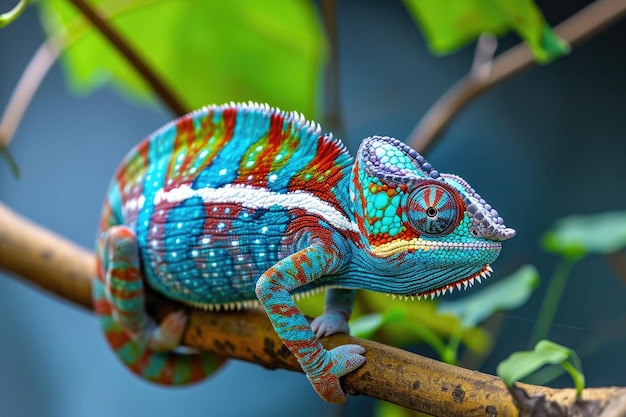The image showcases an absolutely stunning iguana, perched on a tree branch with varying shades of brown and spots. This iguana captivates with a dazzling array of colors, making it perhaps one of the most vibrant animals ever seen. Its primary color is a gorgeous turquoise, with red running through its body and eye-catching turquoise and red lines accentuating its eyes. The iguana’s head and arms are adorned with striking purple and red hues, while its chin is pure turquoise. A distinctive red line, interspersed with white upside-down triangles, runs from its mouth to the tip of its tail. The tail itself mirrors the brilliant turquoise and red color scheme. The iguana, with its unique shading and marking, seems almost chameleon-like and of medium size, tightly grips the tree branch. The background is a blur of dark blue and teal shades, punctuated by hints of green leaves, suggesting that the iguana is outdoors.